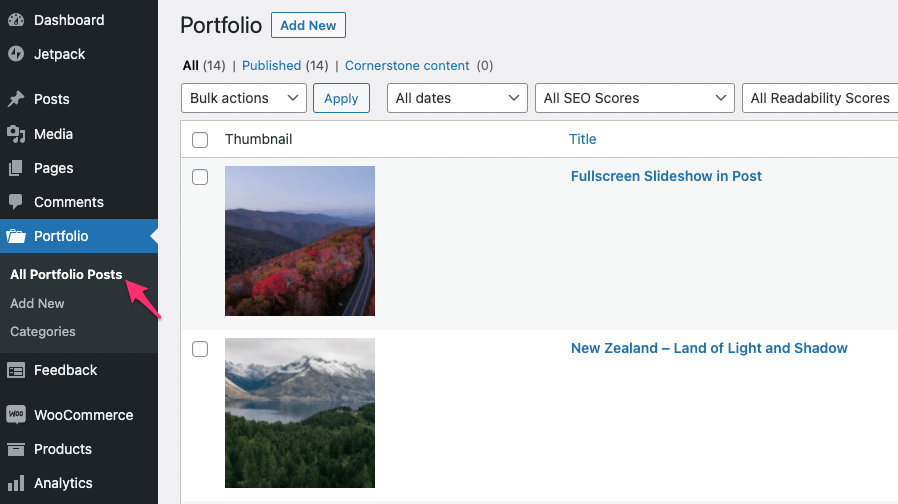This screenshot showcases the interface of a program or a backend website, potentially called Jetpack. On the left side of the image, there's a vertical navigation menu with several options: Dashboard, Jetpack, Posts, Media, Pages, Portfolio, Feedback, WooCommerce, Products, and Analytics. Some of these options, such as Portfolio, are expanded, revealing sub-options like All Portfolio Posts, Add New, and Categories. 

To the right of the navigation menu, the main content area displays Portfolio-related functionalities. At the top, there's an Add New button, followed by filter options labeled All (14), Published (14), and Cornerstone Content (0). Further options include Bulk Actions, Apply, All Dates, All SEO Scores, and All Readability Scores, providing various tools for content management.

The content area also features two images of mountains. One image captures a mountain view from a high vantage point, while the other shows a mountain from the ground level. They are labeled "Full Screen Slideshow and Posts" and "New Zealand Land of Light and Shadow" respectively, hinting that this platform might be used for blogging or selling prints. The interface primarily utilizes a white background with blue and black text, making for a clean and professional appearance.